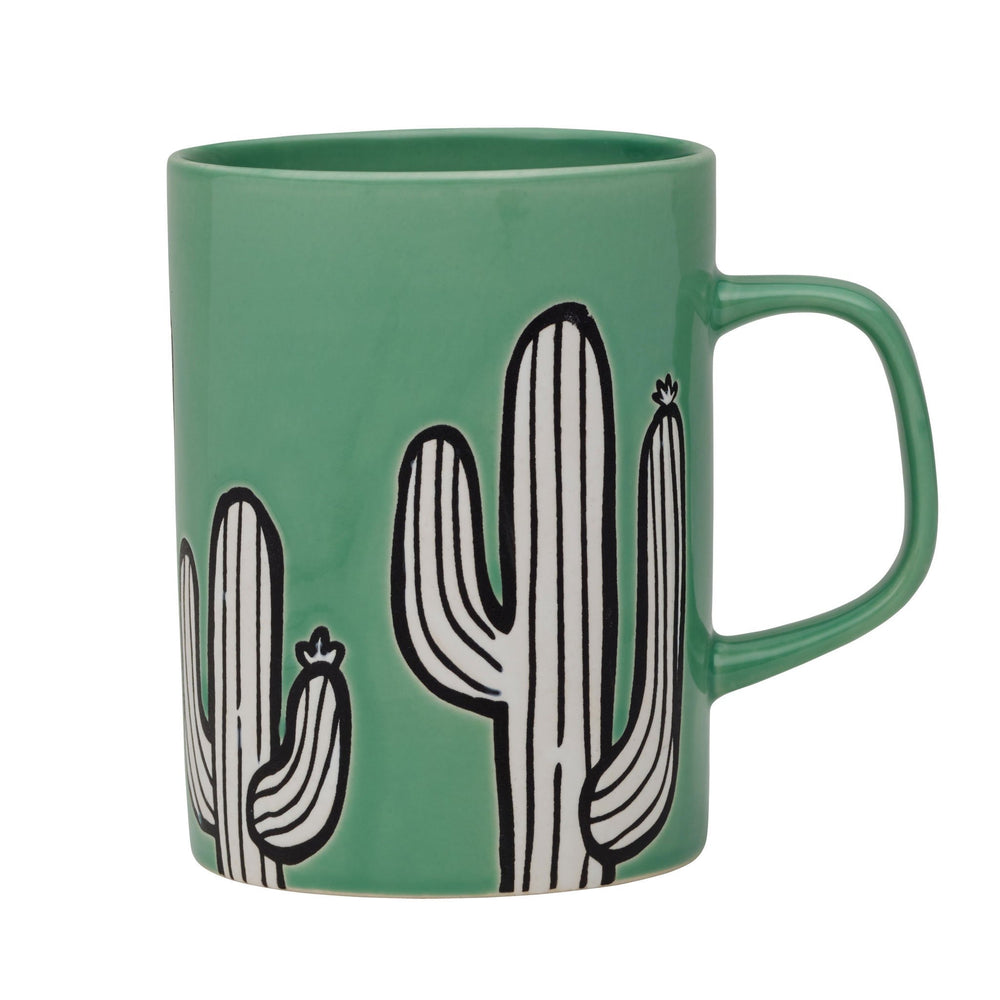The image shows a light mint green coffee mug featuring two white saguaro cactuses with thick black outlines, depicted on a plain white background. The left cactus is shorter while the right one is noticeably taller. Both cactuses have vertical lines across their trunks and branches, adding texture and detail. Small, stylized flowers bloom at the tips of their rightmost arms. The mug has a distinctive handle, with the bottom part extending further out than the top part. The mug is empty and appears to be a standard size, presented as a stock image.